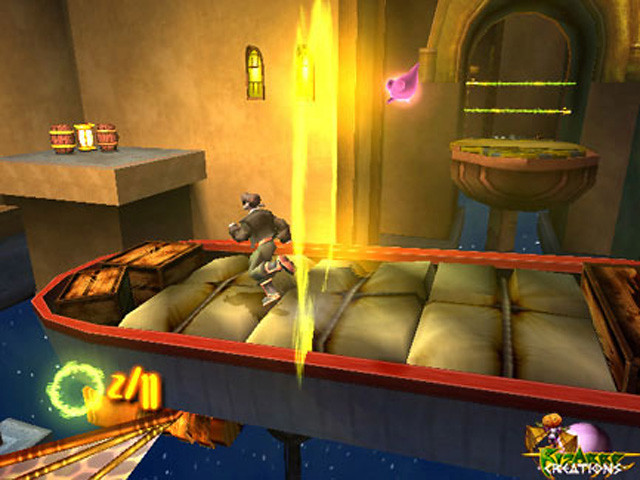In this highly realistic video game screenshot, we see a vibrant and immersive space-themed universe. In the top left corner, an alcove houses a square-shaped platform supporting three wooden barrels, which suggest a storage area for supplies. The main focus of the image is a dynamic character sprinting across a docked spacecraft, suggesting a sense of urgency or action. This character has just passed through a glowing, fiery archway, adding a mystical or intense element to the scene. In the background, the endless expanse of space is beautifully illustrated with a deep blue color palette, dotted with sparkling stars that enhance the otherworldly atmosphere. At the bottom of the image, the numbers "2-11" are visible, possibly indicating a level or a checkpoint within the game. This captivating scene masterfully blends elements of adventure, mystery, and space exploration.